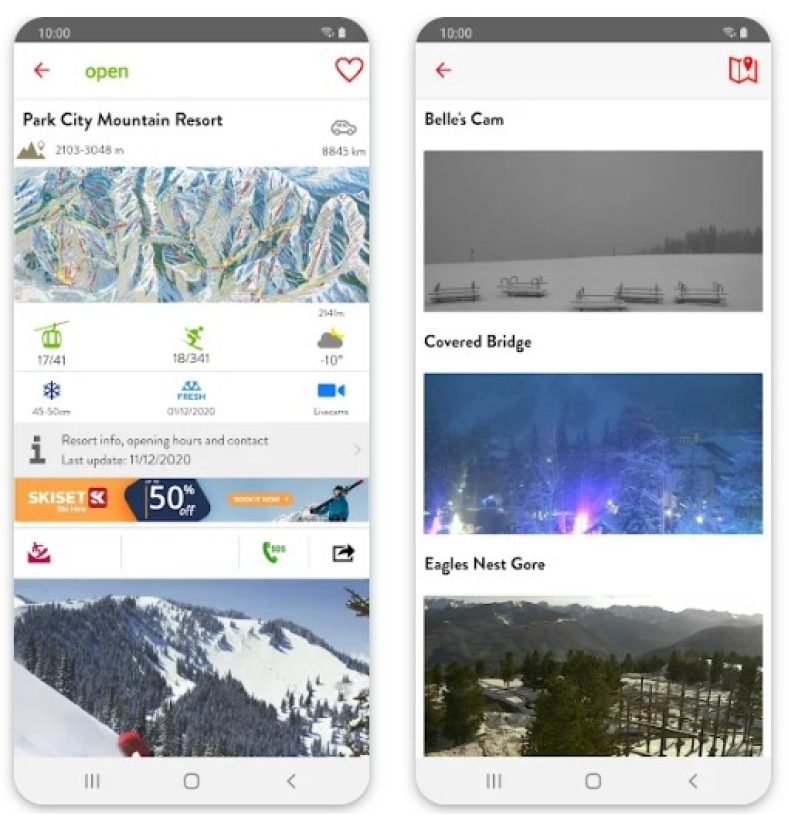The image showcases two different phone screens side by side, each depicting various aspects of a ski resort.

On the left, the phone screen displays a comprehensive layout starting with a gray status bar at the top showing the time as 10 o'clock. The background of this screen is primarily white, accentuated by a green button labeled "Open." Adjacent to this is an icon of a red heart outlined in red with a white interior. Below the heart, in bold black text, it reads "Park City Mountain Resort." Further down, there's a detailed map of a ski mountain, providing an overview of the slopes and trails. At the very bottom of the screen, there is an image of a skier navigating a snowy mountain, capturing the essence of winter sports.

To the right, the second phone screen presents three distinct images, each accompanied by labels. At the top, the text "Bell's Cam" is clearly marked in black, followed by "Covered Bridge" and "Eagle's Nest Gore." The uppermost picture displays a snowy landscape featuring metal benches and chairs under a gray sky, with a backdrop of trees. The middle image captures snow-laden trees illuminated by bright lights, evoking a serene, wintry ambiance. The bottom picture offers a panoramic view of distant, snow-covered mountains with an array of closer trees and tall posts in the foreground, all contributing to the picturesque and tranquil winter setting.